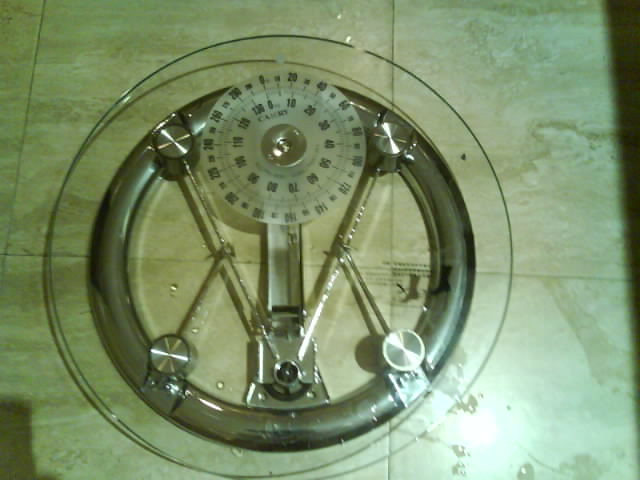This image depicts an old-fashioned mechanical scale situated on a yellowish-green, tiled countertop. The primary focus is a round dial, likely made of glass, which encases a smaller metal circle. Within this metal circle are intricate mechanical connections. The upper portion of the device features a circular gauge with numbers ranging from 0 to 120, suggesting it's a weight scale. The gauge combines silver and white plastic elements, and a faint image of a foot can be discerned, further affirming its function as a scale. Additionally, a light reflects off the bottom right corner, accentuating the tiled surface of the countertop.